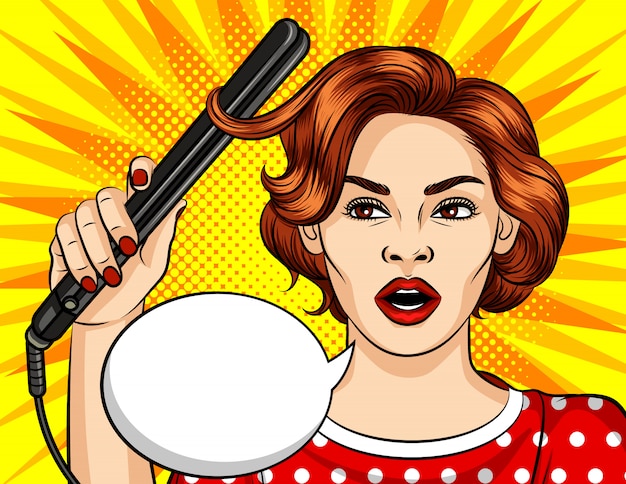The image is a vibrant pop-art style illustration resembling a comic book panel. The background is an animated sunburst with yellow and orange rays, peppered with patterns of dots and geometric shapes. At the forefront stands a woman of European descent with short, wavy auburn hair, styled in a bob. She is working on her hair with a black curling iron held in her right hand, and her red-painted fingernails are visible. The woman's facial features include brown eyes, dark eyebrows, and lips painted with bright red lipstick. She is dressed in a red dress adorned with white polka dots and a white collar. A blank speech bubble hovers near her face, indicating she is about to say something. The overall composition is dynamic, with the vibrant colors and patterns emphasizing the woman's actions and expressions.